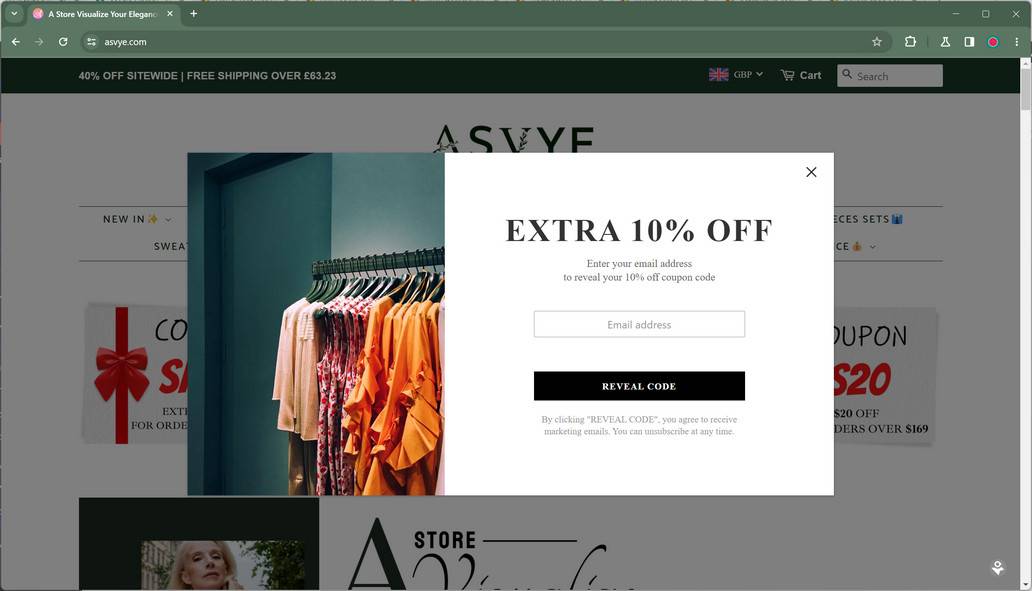This image depicts a retail website page with a focus on elegance, laid out with a clean and inviting interface. At the very top, in a green header with white text, the store's slogan "A Store, Visualize Your Elegance" is prominently displayed. Below this header, there is a navigation bar featuring a back button, a forward button, and a refresh button. The address bar shows the URL "ASVYE.com."

Directly below, there is a dark-colored promotional header announcing "40% Off Site-Wide" and "Free Shipping Over £63 and £23." This section also includes a drop-down menu for currency selection, set to GBP (British Pound), indicated by a British flag icon. To the right of this promotional announcement, there are icons for a shopping cart and a search bar.

The main body of the web page prominently features the store's name, ASVYE, with a visually appealing photograph showcasing a rack filled with an assortment of multicolored blouses and dresses. Additionally, a pop-up box appears in the lower part of the image, offering an "Extra 10% Off" for customers who enter their email address.